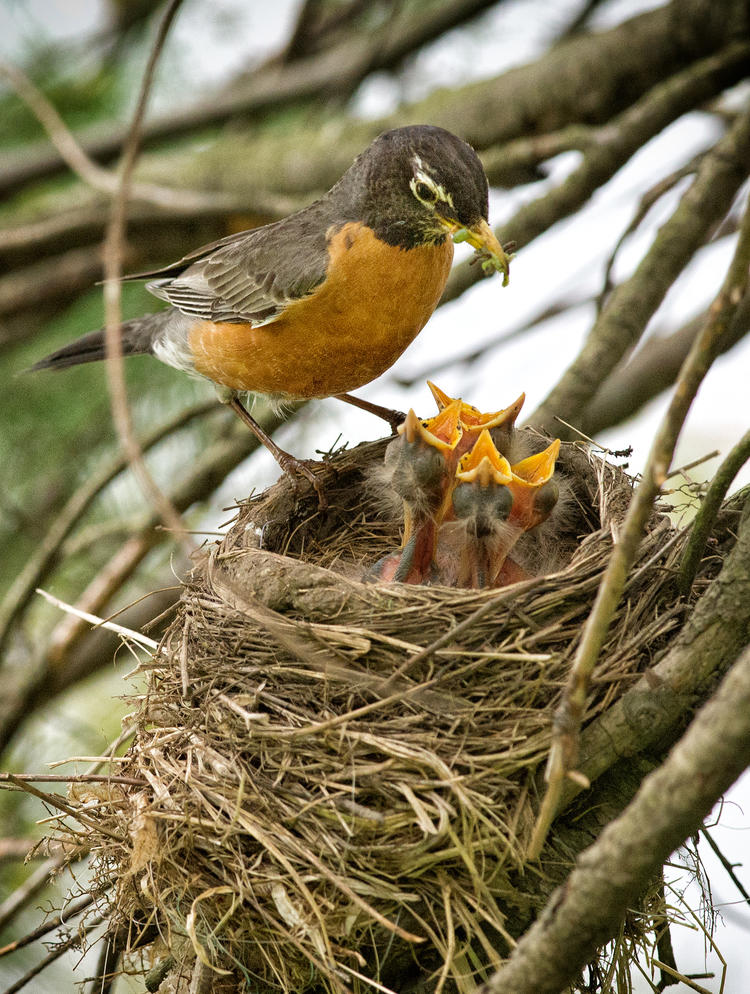This photograph, taken outdoors during the daytime, captures an enchanting moment high in the treetops. The image is rectangular, approximately six inches high and four inches wide, looking up into a network of brown branches that stretch from the upper right to the lower left of the frame. A bluish-gray sky peeks through the branches on the right, while the left side is filled with the blur of green leaves, suggesting the photograph was taken in a season other than winter.

At the bottom center of the photo, there's a meticulously constructed bird's nest made of light tan straws, dead grasses, and bits of fur. The heartwarming focal point of the image is the four baby birds nestled inside the nest. These chicks have gray bodies with a touch of red and sparse tufts of white feathers, appearing almost hairless. All four of them have their orange beaks wide open, eagerly waiting to be fed.

Perched on the upper left edge of the nest is the adult bird, likely a robin, with distinct characteristics including a dark brown head and back, a rich red chest, a yellow beak, and white around its eyes. The robin is caught in the act of feeding its young, holding small green bugs in its beak, ready to drop them into the wide-open mouths below. The scene paints a beautiful and detailed portrait of nature, showcasing the intimate feeding ritual of a robin and its chicks.